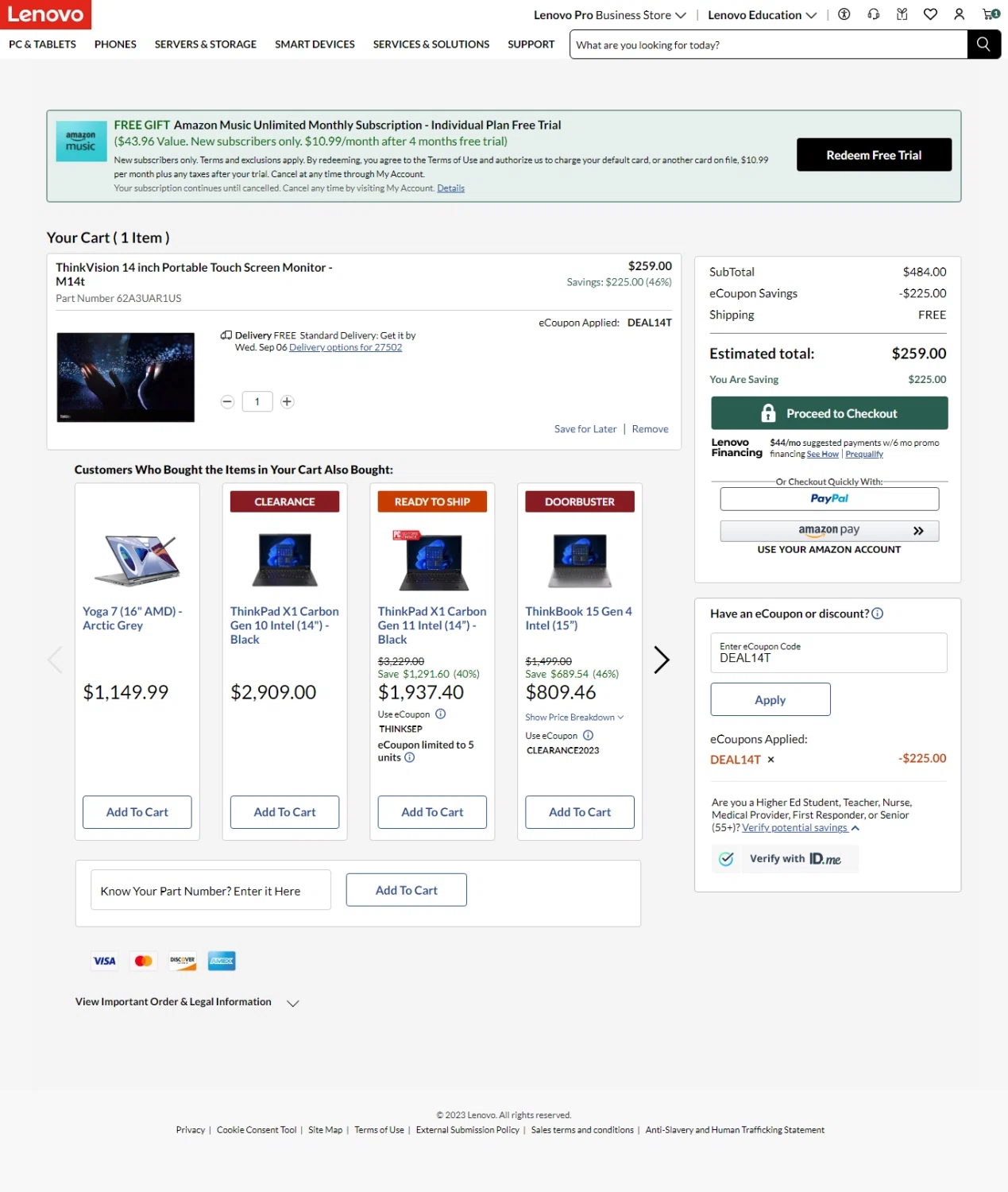This image is a screenshot from the Lenovo website, showcasing various aspects of the online shopping experience. In the upper left corner, the Lenovo logo is prominently displayed inside a red rectangular box with white lettering. Below this, there is a navigation menu with clickable categories including "PC & Tablets," "Phones," "Servers & Storage," "Smart Devices," "Services & Solutions," and "Support."

The main focus of the screenshot is the shopping cart, which contains one item: the "ThinkVision 14-inch Portable Touch Screen Monitor," priced at $259. Surrounding the cart details, there’s a section that reads, "Customers who bought items in your cart also bought," featuring four images of laptops. Each laptop is situated within white vertical boxes, accompanied by their respective prices and additional tags such as "Clearance," "Ready to Ship," and "Door Buster." Each of these laptops has an "Add to Cart" button below it.

To the right of the cart summary, there’s a breakdown of costs, including the item subtotal, coupon savings, free shipping, and an estimated total of $259. Below this summary, there’s a green rectangular "Proceed to Checkout" button with a lock icon, as well as options to pay through PayPal and Amazon Pay. The lower section of the screenshot includes various text elements and pictures which are not clearly readable.